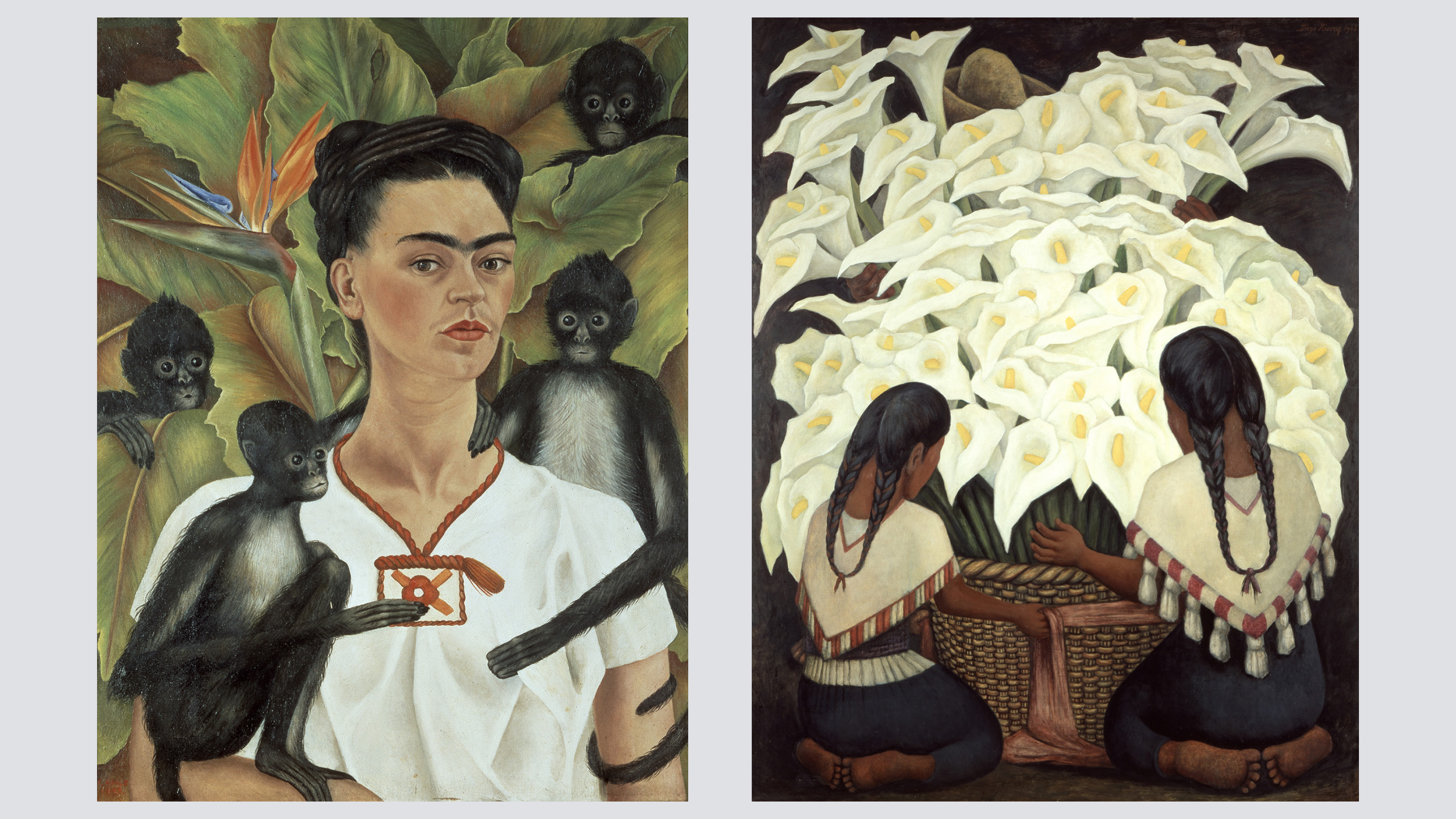In an art museum, two captivating paintings hang side by side. The left painting is a detailed portrait of Frida Kahlo, distinguished by her characteristic arched eyebrows and dark hair elegantly piled on top of her head. She is dressed in a pristine white shirt and is surrounded by a lively troupe of monkeys. One monkey is perched comfortably on her forearm, another clings to her shoulder, while others playfully navigate through the large, lush fronds of a plant behind her. 

The painting on the right depicts a serene scene of two young girls, who appear to be of Native American or Indio descent. They are kneeling on cushions beside a large reed basket brimming with vibrant white flowers, each flower bearing a distinctive cup shape. Behind the girls, a sombrero peeks out from the lush greenery, adding a touch of cultural authenticity. Both paintings, rich in color and detail, capture intimate moments with striking clarity, making them compelling pieces in the museum's collection.